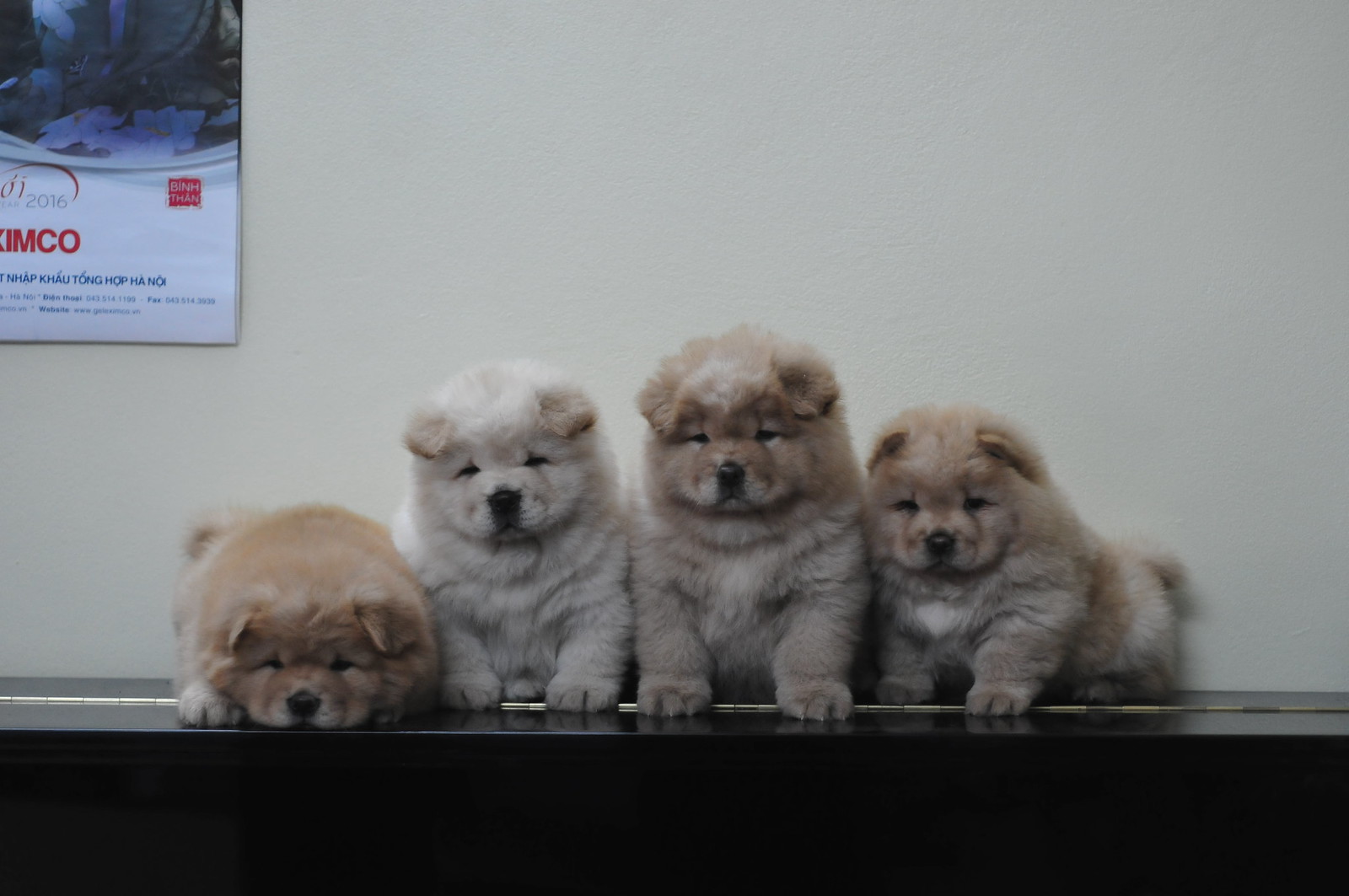Four adorable Chow Chow puppies in varying shades of brown and beige are lined up on a black table, positioned against a white wall. From left to right: the first puppy, a dark brown one, is laying down with its nose at the edge of the table and one white paw visible. The second is a light cream color, sitting upright with darker brown ears and a black nose. The third puppy has a dark brown head and ears, a black nose, and a light brown chest; it's also seated. The fourth stands with a light brown head, dark brown ears, a black nose, and a light brown chest marked with a small white patch. Behind them, slightly out of focus in the top left corner, is a white poster or calendar with red and blue writing, dated 2016. Despite the fuzzy image, it's possibly showcasing a snowy forest scene. The table features a small silver hinge across its center. The setting could be a veterinarian's office or a breeder's home, capturing a moment of sheer puppy cuteness.